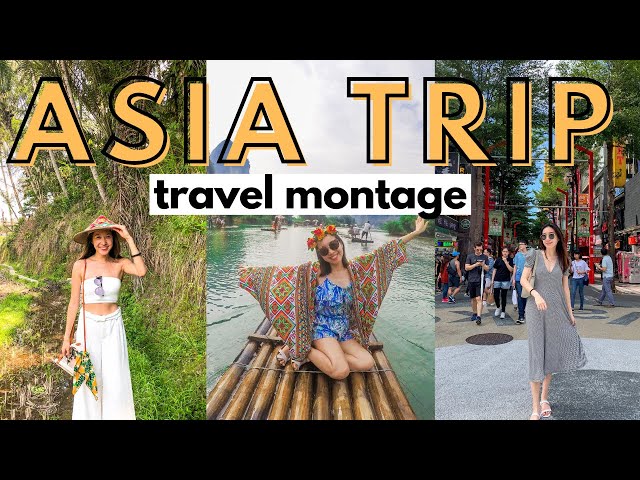The image is a YouTube thumbnail from 2012 or 2014, prominently featuring large yellow letters that read "Asia Trip" and below that, "Travel Montage" in black letters on a white background. It consists of three photos of the same young woman with brown hair, arranged from left to right.

In the first photo on the left, she is standing against a lush, tree-filled backdrop reminiscent of a jungle. She is dressed in an elegant white skirt and top adorned with floral patterns, accessorized with a wide, woven hat and a white purse that has a yellowish-green handkerchief hanging out. Purple sunglasses are tucked between her top. She is smiling warmly.

The center photo shows her kneeling on a simple wooden raft on a river, surrounded by water and other people on similar rafts in the background. She is wearing a light blue jumper with a decorative, multicolored kimono-type jacket over it. She has flowers on her head and wears sunglasses, extending her arms outward in a joyful pose, smiling happily.

In the final photo on the right, she is donning a stylish gray dress and sunglasses while standing on a busy city street. The background features buildings and numerous people walking around, creating an urban scene. While she appears to be smiling in this photo as well, it is less clear than in the others.